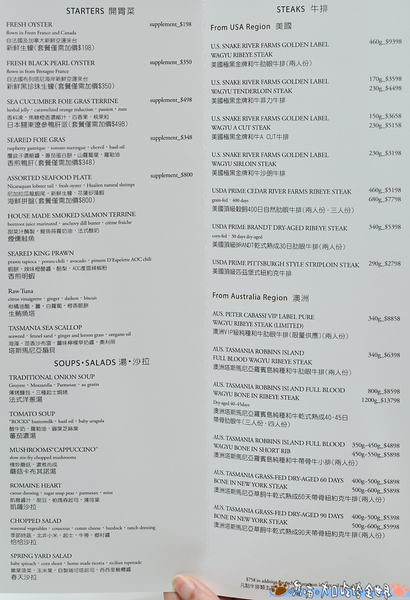The image shows a close-up of a menu, photographed on white paper that appears grayish in the picture. A hand is visible at the bottom right corner, with two fingers delicately holding the menu in place. The menu features blue and black text, with the blue writing less prominent and the black text mostly in an Asian script. 

On the right-hand side of the menu, the section labeled "Steaks" is followed by details listed in an Asian language, along with the phrase "from USA region." Below this header, there are seven individual selections, each accompanied by its price. Further down, another subheading reads "from Australia region" followed by more Asian text and six individual selections with their corresponding prices.

The left-hand side of the menu starts with the section titled "Starters" with its listings in an Asian language. This section includes nine different options. Underneath, another section labeled "Soups & Salads" includes both text in Asian script and a list of six items. Each section presents its items in a structured arrangement, making the menu comprehensive despite the small, difficult-to-read text.